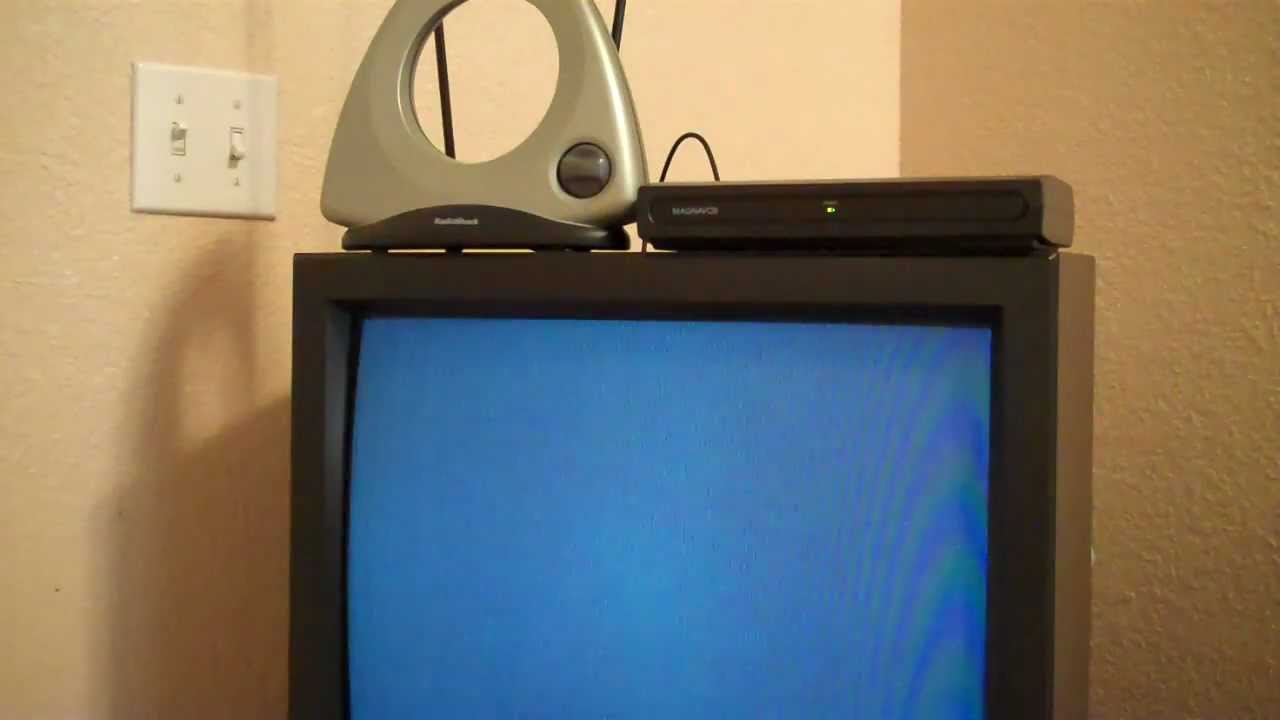The image features an old cathode ray tube (CRT) television with a black square frame, situated in the corner of a room where the walls meet. The screen displays the familiar gray fuzz of static. Positioned on top of the TV are a black DVD player and a TV antenna with two long, black ears. Beside the DVD player is an intriguing electrical gadget shaped like a triangle with a circular cutout, featuring a knob on the bottom right corner. On the left wall, two electrical switches are visible; one is flipped up, the other down. The walls in the background are painted a very light shade that appears either brown or lavender, adding a nostalgic ambiance to the scene.